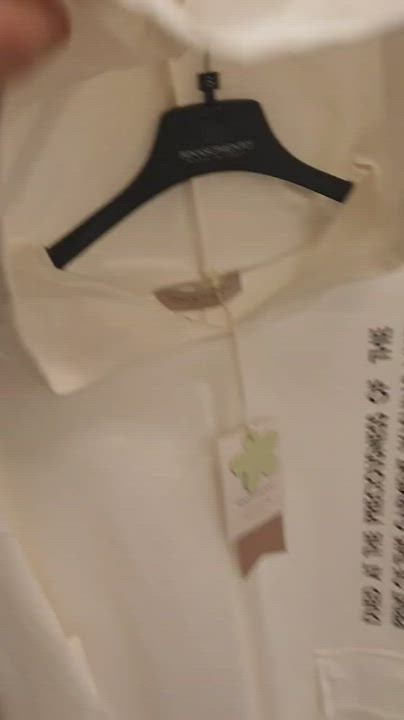This is a detailed photograph of a white shirt on a black hanger. The shirt features a pointy, downward-pointing collar with the right side slightly bent up. There is a pocket on the left side of the shirt's chest, and some blurred writing on or near the pocket. The hanger is black with an indiscernible printed marking on it, and only the upper portion, including the hook, is visible. At the back of the collar, there is a brownish-gray tag, from which a thin string hangs. Attached to the string is a white tag with a brown bottom and a green flower shape on it. The shirt appears new, given the presence of these tags. The image is somewhat blurry and has additional blurred text along the right side. There is also a barely visible human thumb in the upper left corner, possibly holding onto the shirt or hanger. The background is white, providing a stark contrast to the shirt and hanger.